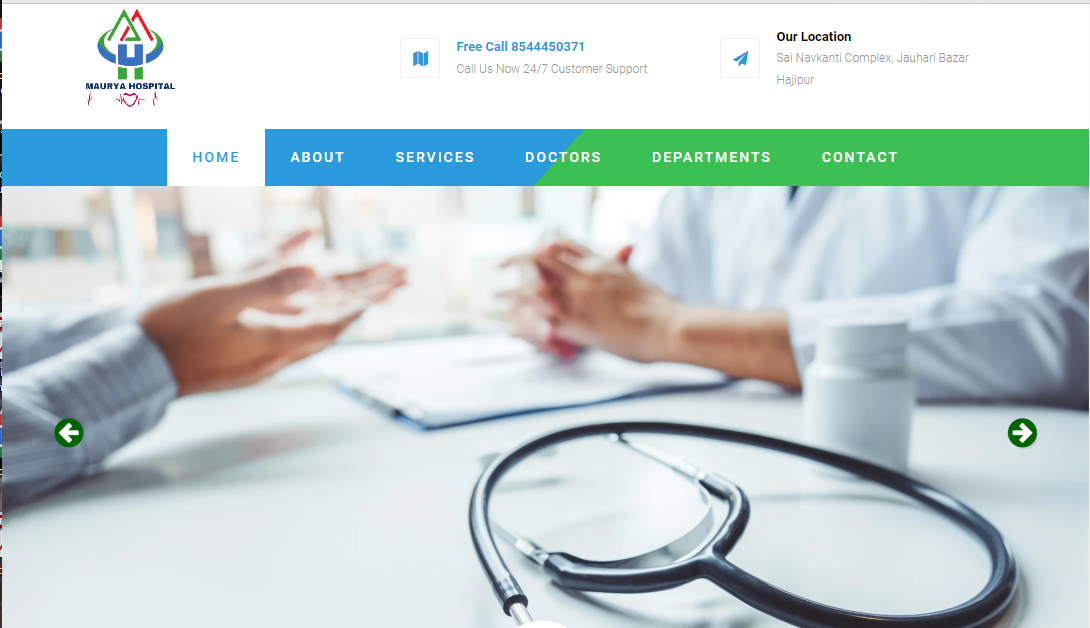This image showcases the homepage of the Maria Maurya Hospital website. The top section of the website features a clean white background. Prominently displayed at the top is the name "Maria M-A-U-R-Y-A Hospital," with a hospital logo above it and a heart symbol below. The logo consists of a green and red "M" and a blue and green "H," encircled by a ring. 

To the right of the logo, centered, is a section offering a "Free Call" service, accompanied by a phone number and a note stating "Call us now - 24/7 customer support." Further to the right, the website lists the hospital's location under a header labeled "Our Location."

Beneath this header is a navigation bar colored half blue and half green, with tabs for various sections of the website, including Home, About, Services, Doctors, Departments, and Contact. Below this navigation bar, the main section of the homepage displays an image of a doctor and a patient engaged in a conversation. The doctor is holding an open chart or folder, and on the table in front of them are a stethoscope and several pill bottles. The overall design of the website appears intuitive and user-friendly, providing easy access to crucial information and resources.